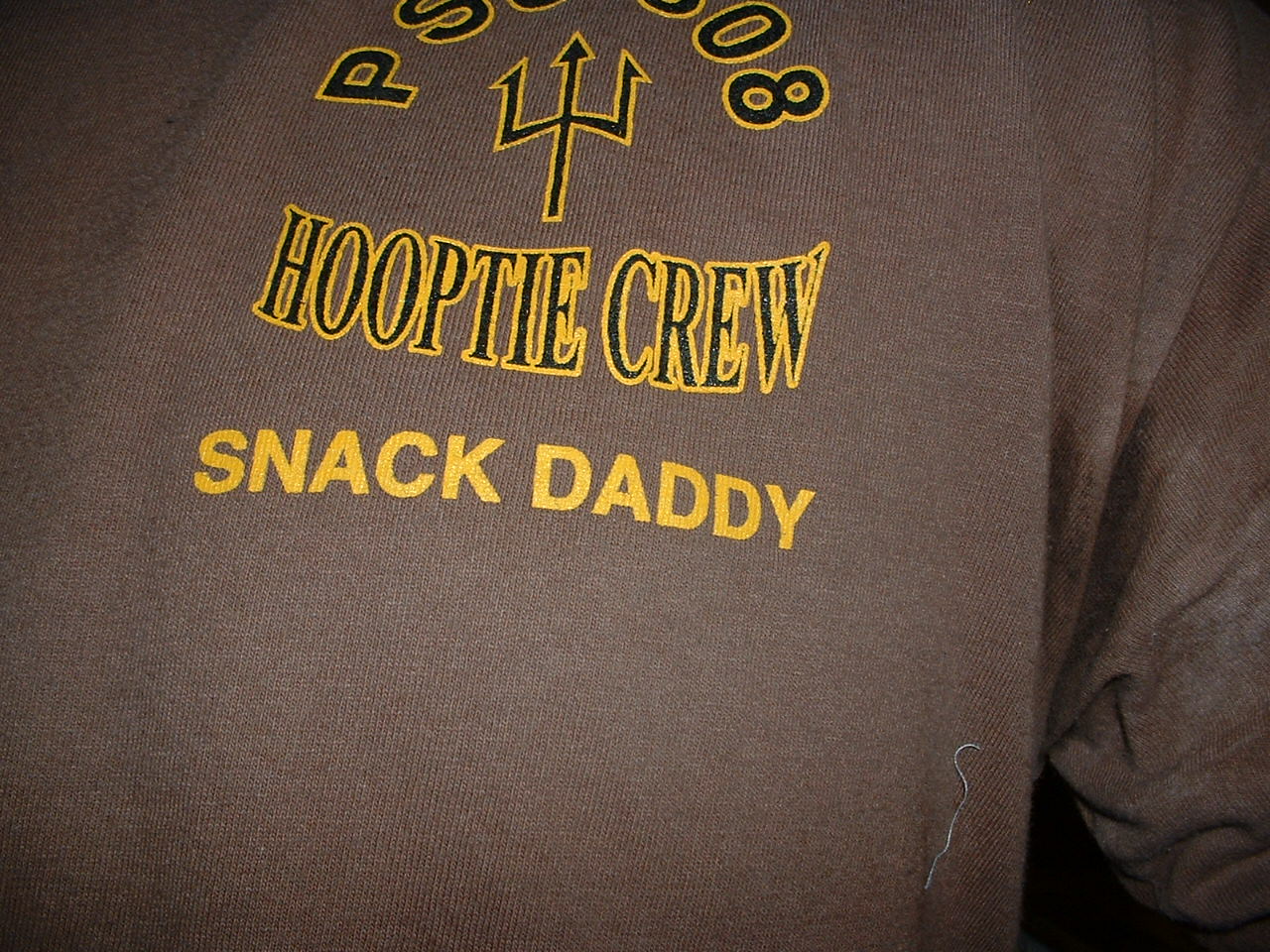This close-up image showcases a male wearing a light eggplant-colored, long-sleeved shirt. The fabric of the shirt appears slightly ribbed. Prominently featured in black letters outlined in gold are the initials "PS" followed by the number "08," though the middle portion of the text is obscured. Below the text, a black trident symbol, also outlined in yellow, is visible. Beneath the trident, the inscription "Hoopty Crew" is written in black capital letters with a yellow outline. Further down, "Snack Daddy" is displayed in yellow capital letters. A light blue thread is stuck to the bottom of the shirt. The background of the image is predominantly black, with some shadowy areas visible between the person's torso and upper arm.